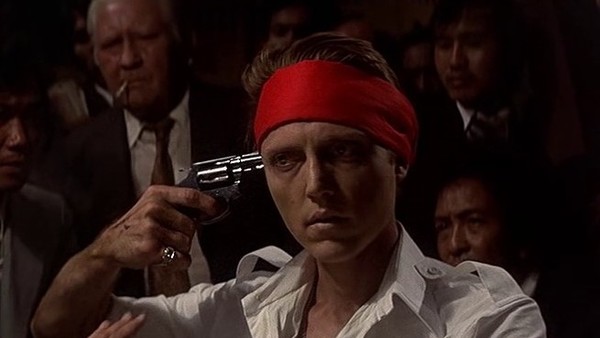This image is a still from an older movie, featuring a young Christopher Walken at its center. Walken, wearing a white dress shirt open at the neck and a red headband that holds back his brownish hair, has a serious expression as he holds a pistol to his temple with his right hand. A diamond pinky ring can be seen on the same hand. The color photograph has a slightly off-tone quality, typical of films from past decades. In the background, several blurred figures can be seen, predominantly Asian men. To Walken's left, an older gentleman with white hair stands out clearly. This man is adorned in a dark suit, brown tie, and white collared shirt, smoking a cigarette. Another partially visible person, also appearing to be Asian, is slightly off the screen to the left. The image evokes a dramatic and intense atmosphere, capturing a poignant cinematic moment.